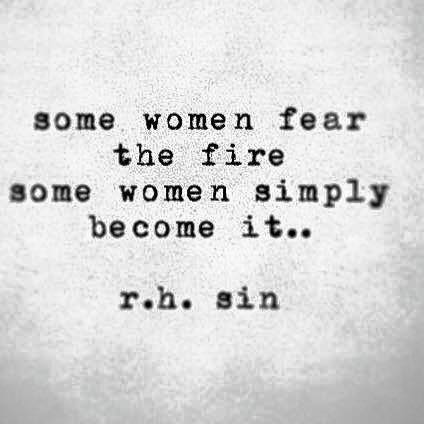The image depicts a texture of aged white paper, speckled with small gray blotches suggesting a worn, vintage quality. A typewritten statement is inscribed on the paper, composed entirely in lowercase letters. The text reads: "some women fare the fire. some women simply become it.." and is arranged across four lines. The first line contains "some women fare," the second line reads "the fire," the third line states "some women simply," and the fourth line concludes with "become it.." The statement is followed by a skipped line, beneath which the author's name, "rhsin," appears, also in lowercase letters. The text is generally centered on the page but leans slightly to the left, maintaining a balance both horizontally and vertically.